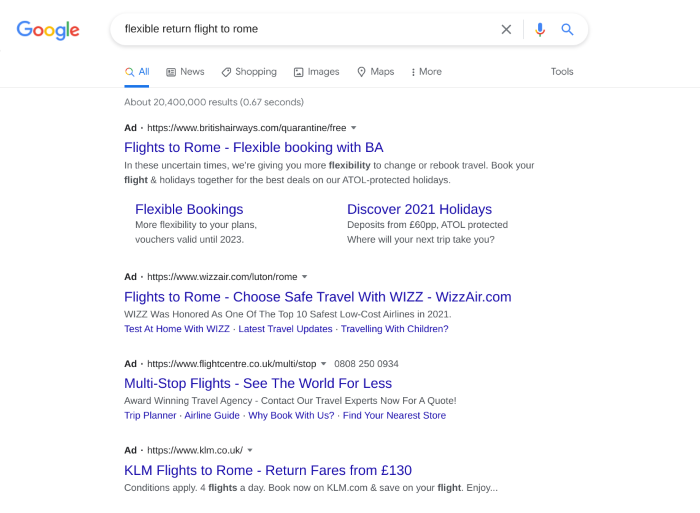The image depicts a webpage displaying Google search results for the query "flexible return flight to Rome." In the upper left corner, the iconic multi-colored Google logo is prominently visible. To the right of the logo, there is a search bar displaying the queried text with attached icons: a gray 'X' for clearing the search, a microphone for voice search, and a magnifying glass symbolizing the search function.

Below the search bar, the search results information indicates that approximately 20,400,000 results were retrieved in 0.67 seconds. The list of results consists of four sponsored ads, each marked with a black "Ad" label followed by the respective website addresses.

1. The first ad is from British Airways with the URL "BritishAirways.com/quarantine/free." The blue text beneath reads "Flights to Rome - Flexible booking with BA."
2. The second ad is from Wizz Air, displaying the URL "www.wizzair.com/Luton/Rome," with the description "Flights to Rome - Choose safe travel with Wizz Air."
3. The third ad is from Flight Centre, listed as "flightcenter.co.uk."
4. The final ad is from KLM with the URL "www.klm.co.uk."